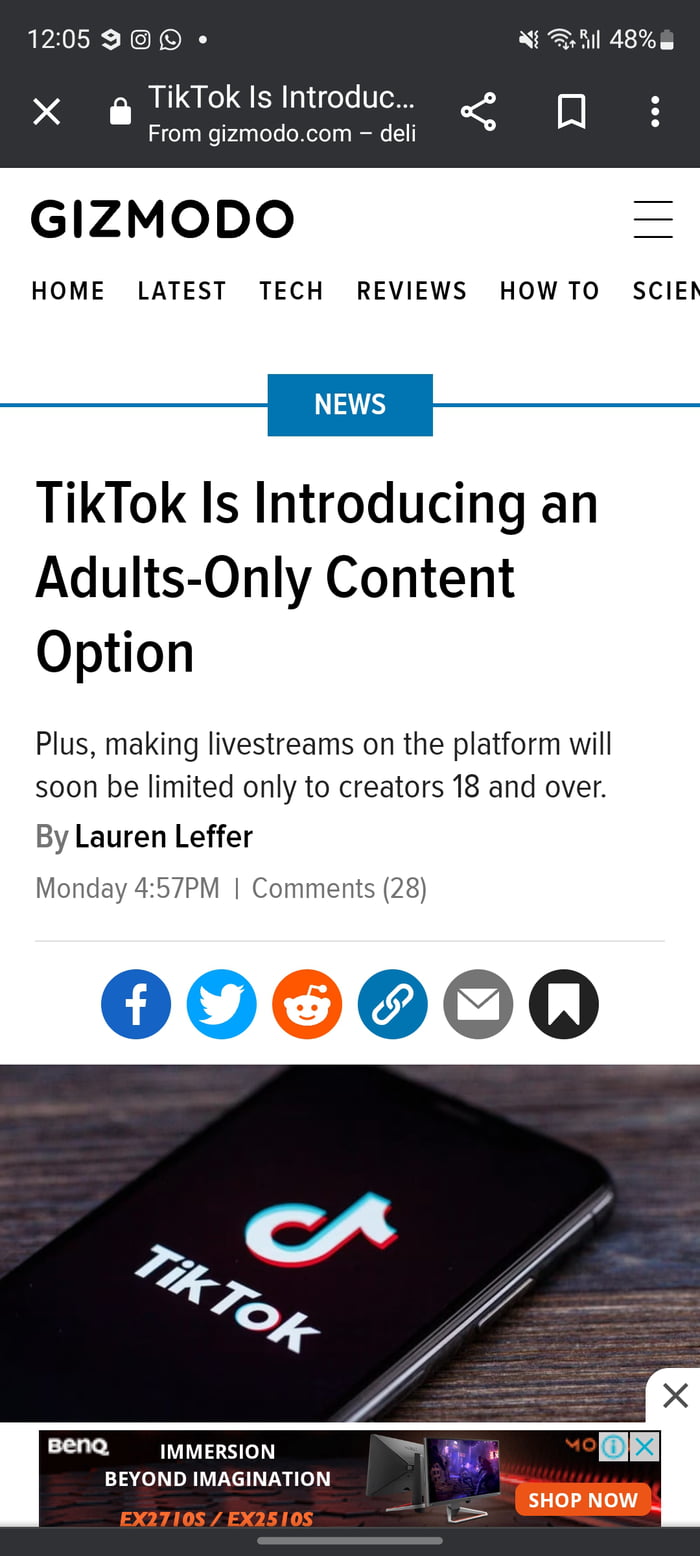The image depicts a digital screen with a mobile interface, segmented into various sections. At the top of the screen, there is a gray and white status bar displaying the time "12:05" on the left, and an Instagram camera icon. Next to it, there's a white WhatsApp icon. To the right, it shows a battery level icon indicating 48% in white, suggesting the battery is less than half full.

Directly below the status bar, on the next row, there is a white "X" icon on the left-hand side and a white lock icon. In this row, white text reads "TikTok is introduced," which ends abruptly with a cut-off "C" followed by an ellipsis (…). Beneath this partial text, more white text reveals "from Gizmodo.com/deli."

The background turns white, and on the left-hand side, the word "Gizmodo" appears in black font. On the right-hand side, there are three black horizontal lines indicating a menu. Below this section, a series of black text lists site navigation options: "Home, Latest Tech Reviews, How To, SCIE," with the last word cut off.

A blue rectangle spans the width of the screen, with "News" written in white inside it. A horizontal line extends from this rectangle to both the left and right edges of the screen.

Further down in black text, the headline reads: "TikTok is introducing an adults-only content option. Plus making live streams on the platform will soon be limited to creators 18 and older," authored by Lauren Leffer. Below this in gray text, it says "Monday 4:57 PM," with "comments 28" following.

At the bottom of the image, there is a visual showing a black smartphone displaying the TikTok app. The phone is placed on a wooden surface, rounding out the lower section of the screen.